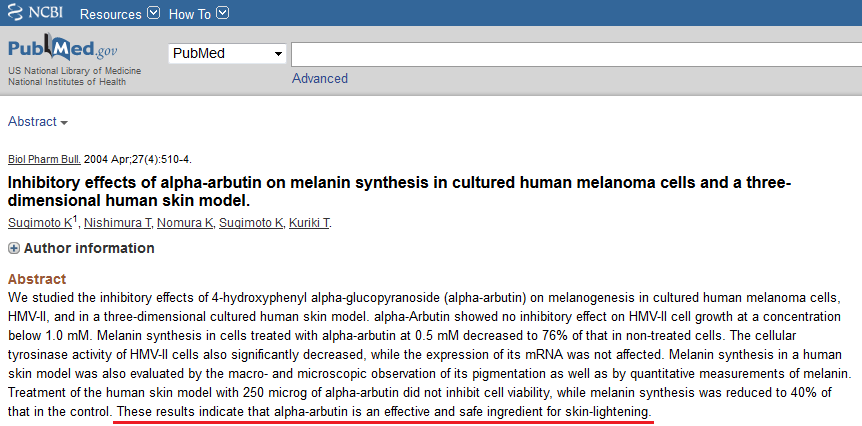The image depicts a webpage from the National Center for Biotechnology Information (NCBI). At the top of the page, the NCBI logo featuring wavy lines is prominently displayed. Next to the logo, the acronym "NCBI" is clearly visible. The blue header bar beneath the logo contains several elements: a resource link indicated by a downward-pointing arrow enclosed in a box, another similar box also pointing downward labeled "how-to."

Below the header, the page prominently features "PubMed.gov." Directly below this, there is a category option box related to PubMed, followed by a search bar, with an "Advanced" link positioned underneath the search bar. Adjacent to the "PubMed.gov" site identifier is a listing for the U.S. National Library of Medicine and the National Institutes of Health.

Further down, the page transitions into an abstract view with an upside-down triangle indicating expandable categories. Listed is a reference to a scientific article titled "BioPharm Bull, 2004 April 27(4):510-4.0," focusing on the inhibitory effects of alpha-arbutin on melanin synthesis in cultured human melanoma cells and a three-dimensional human skin model. Below the article title, the authors are listed, each with a clickable link directing to their profiles or contributions.

The abstract of the article is then provided, summarizing the research. A noteworthy result highlighted in the abstract reads: "These results indicate that alpha-arbutin is an effective and safe ingredient for skin lightening," with the entire sentence distinctly underlined and highlighted in red, emphasizing its importance.